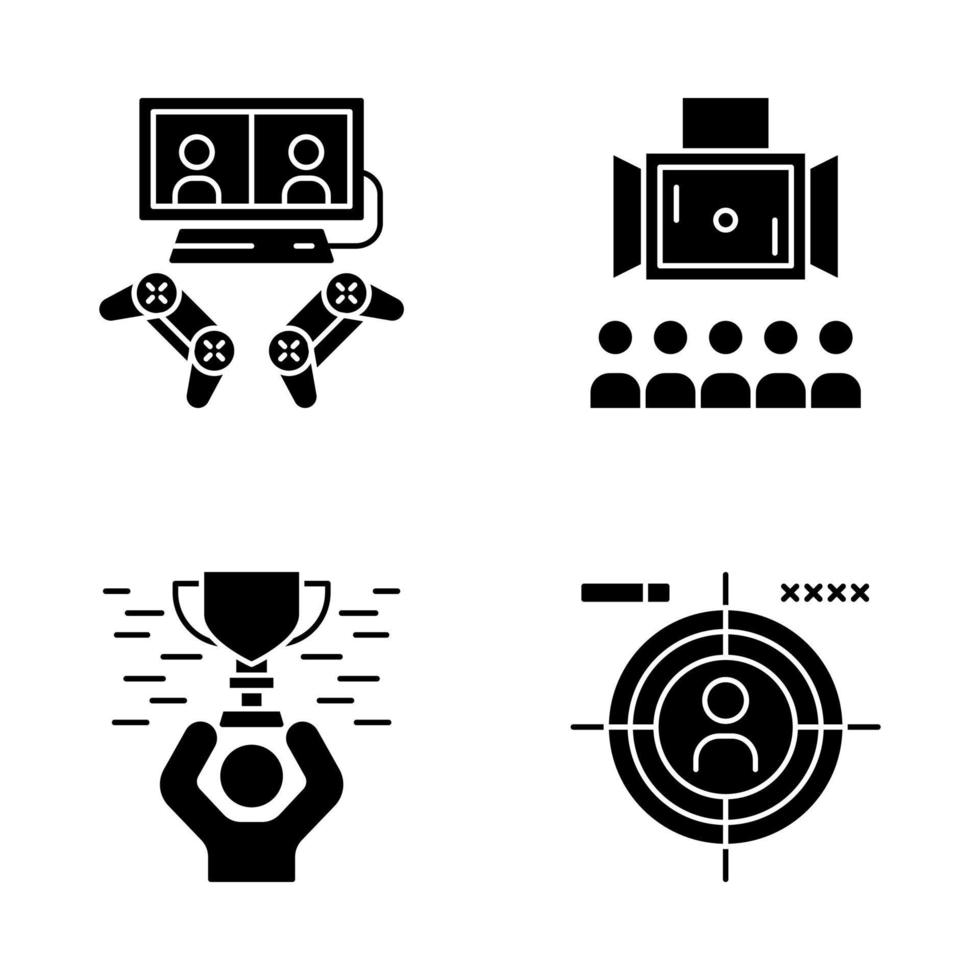This digital image features four black-and-white icons arranged on a minimalist white background. In the top left, there's a simplistic depiction of a TV with two stick-figure heads on either side, connected to a console below it, which has two wireless controllers underneath. The top right icon displays a black rectangular box with a white circle in the middle, flanked by vertical lines on either side, reminiscent of a Pong game setup. Below this box are five player icons, indicating multiplayer capability. The bottom left corner shows a stick figure holding up a trophy, signifying victory or achievement. Finally, the bottom right icon portrays a bullseye target with a human form in the center, accompanied by a health bar at the top left and four X's at the top right, suggesting a targeting or combat scenario. Each icon is rendered in a simple, textureless silhouette, emphasizing a clean and straightforward design.